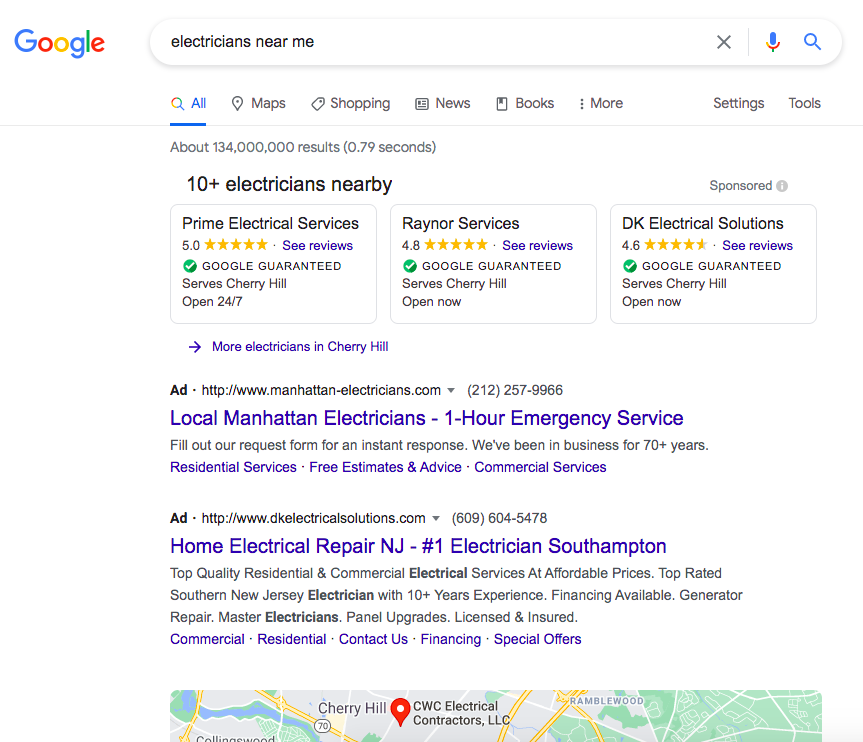The image showcases a Google search page where someone is looking for local electricians. The familiar Google logo is positioned at the top left, next to a search bar with the query "electricians near me." On the right side of the search bar are an "X" icon for clearing the search, a microphone icon for voice search, and a magnifying glass icon for initiating the search. Below the search bar, there are filters for different types of search results: All, Maps, Shopping, News, Books, More, Settings, and Tools. The "All" tab is the active filter, highlighted in blue and underlined, while the rest are gray.

The results indicate about 134 million findings in 0.79 seconds. The listing begins with a highlighted section that states "10+ electricians nearby," featuring three prominent entries displayed in boxes: Prime Electrical Services, Rainer Services, and DK Electrical Solutions. 

- **Prime Electrical Services** has a 5-star rating, is Google Guaranteed, serves Cherry Hill, and operates 24/7.
- **Rainer Services** has a 4.8-star rating, is also Google Guaranteed, serves Cherry Hill, and is currently open.
- **DK Electrical Solutions** has a 4.6-star rating, is Google Guaranteed, serves Cherry Hill, and is currently open.

Below this section, there’s a link offering to show more electricians in Cherry Hill. Following this, two advertisements are featured:

1. An ad for local Manhattan electricians, promoting a one-hour emergency service.
2. An ad for Home Electrical Repair in New Jersey, claiming to be the number one electrician in Southampton.

The detailed nature of the search results offers users a quick comparison of available services and their ratings, operational hours, and other essential details.